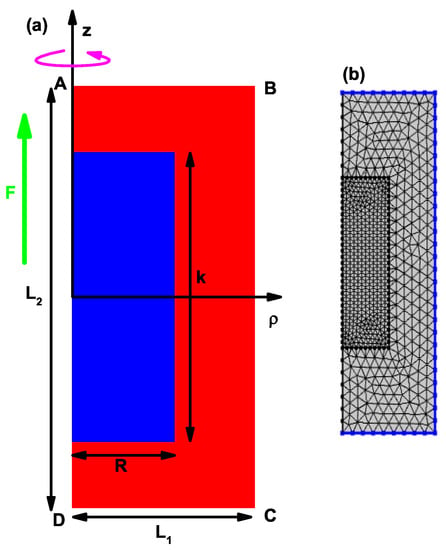The image is a detailed mathematical diagram explaining shapes and their dimensions, prominently featuring two main rectangles. On the left side, there's a larger red rectangle with a smaller blue rectangle inset within it. The red rectangle is labeled with a capital "B", while the inset blue rectangle includes arrows pointing in multiple directions. A black arrow points left and right and is labeled "R," whereas another black arrow points up and down labeled with a lowercase "k." Above these, a green arrow pointing upwards is marked with a capital "F," and a bidirectional black arrow points up and down, labeled with both "A" (on the top end) and "D" (on the bottom end). Below this setup, a horizontal arrow labeled "L1" has arrowheads on each side labeled "D" and "C."

On the right side of the diagram, another rectangle is visible, labeled with lowercase "b" in parentheses. This rectangle features a crisscrossed gray and white pattern and includes a smaller inset rectangle of the same pattern. The detailed geometric pattern of small triangles adds complexity to the design. Additionally, there are intersecting arrows with varied labels such as "A," "L2," "D," "a," and "z" denoting different dimensions and directions.

This amalgamation of labels, arrows, and patterns provides a comprehensive breakdown of the spatial and dimensional relationships within the outlined shapes.